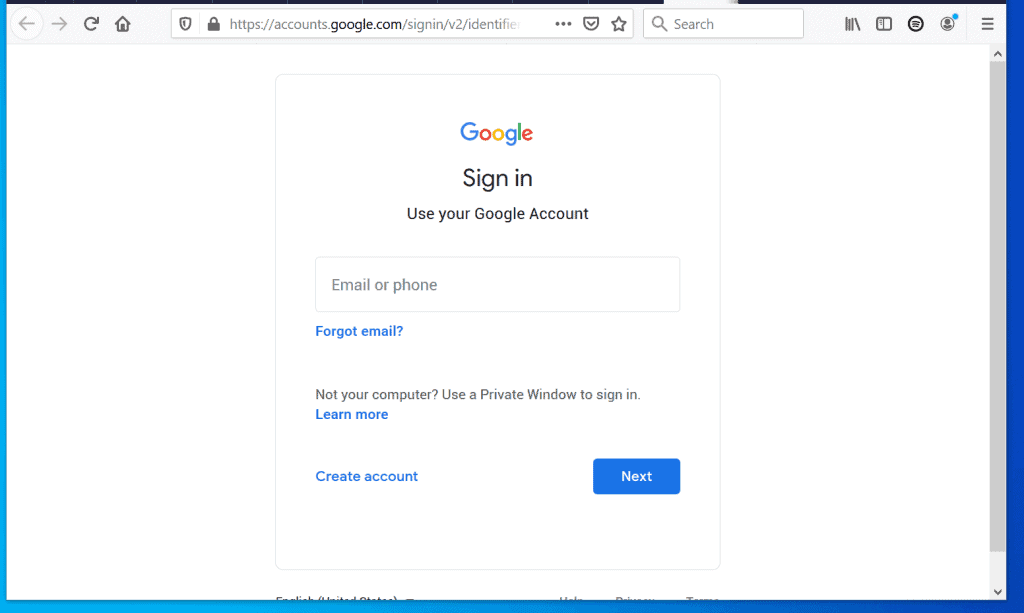A screenshot captures a web browser window navigating to the Google sign-in page. The browser's interface exhibits a predominant white background framed by a very light blue, thin border, likely glimpses of the desktop background. The browser's top bar is grey, showcasing standard navigation icons: a left-pointing arrow, a right-pointing arrow, a circular arrow, a house icon, followed by the address bar. The address bar contains an image of a shield and a lock, displaying the partially cut-off URL "https://accounts.google.com/signin/v2/identify." To the right of the address bar are three horizontal dots, a V-shaped symbol, a star icon, a search box, and various other icons including what appears to be a series of books, an open book, a Spotify widget, an icon of a person within a blue circle, and three vertical lines.

In the main section of the window, the familiar Google logo is centered at the top. Below it, the text "Sign in" is prominently featured, followed by "Use your Google Account." There is an input box labeled "Email or phone" for username entry. A "Forgot email?" link, written in blue, appears under the input box. Beneath this, the text "Not your computer? Use a private window to sign in" is displayed, with "Learn more" in blue text immediately below. At the bottom, the option to "Create account" appears in blue text, beside which a blue button labeled "Next" is positioned on the right-hand side.